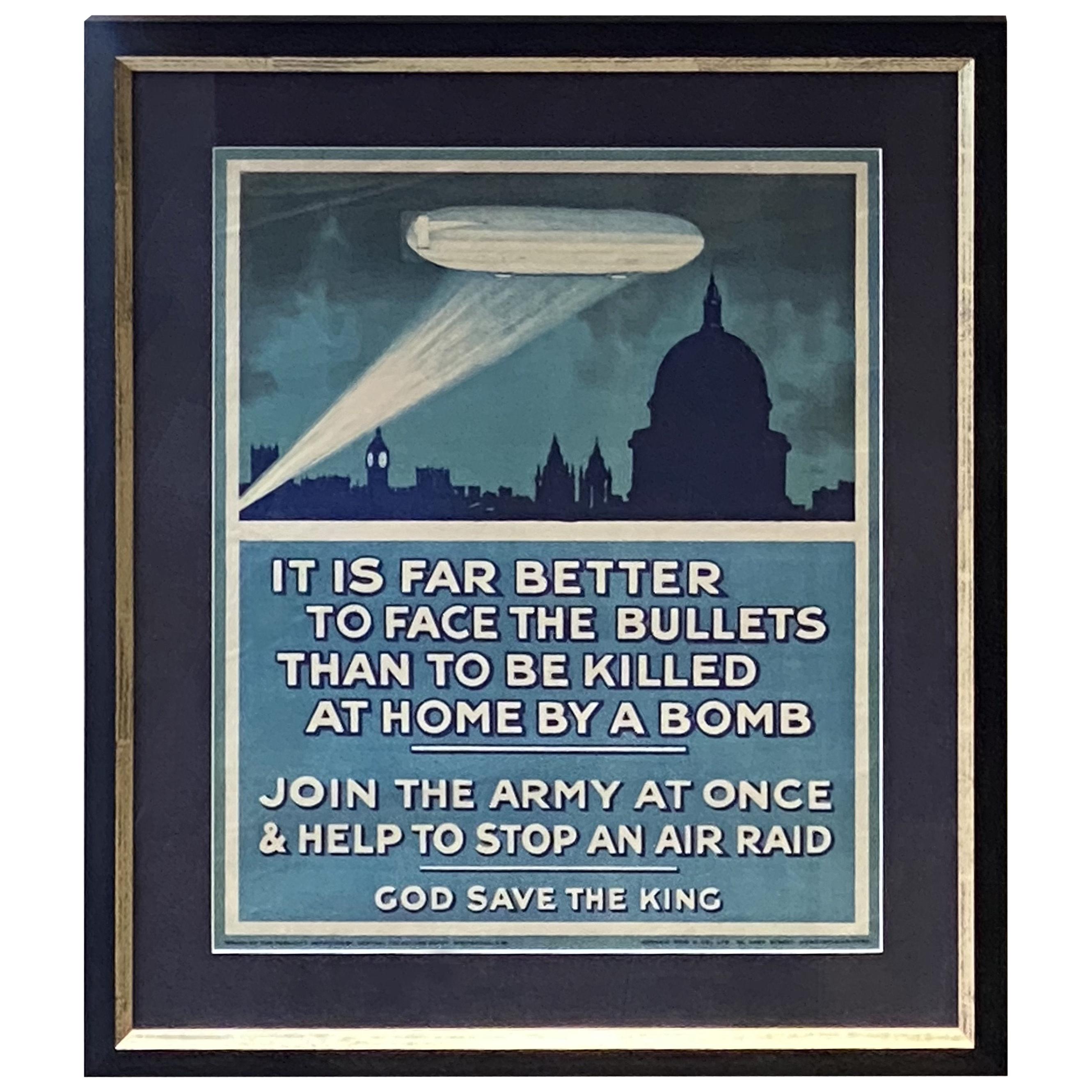This image prominently features a framed, hand-painted illustration set against a black background with a gold-edged, black beveled frame. The inner matte is black with a thin teal edge. The top half of the image depicts a nighttime cityscape with a large dome—resembling the Capitol building or possibly a mosque—on the right, surrounded by smaller buildings. Above the cityscape, a gray blimp is highlighted by a spotlight shining from the bottom left, casting a glow through the dark, cloudy sky. The bottom half of the image contains white text on a blue background, reading: "It is far better to face the bullets than to be killed at home by a bomb. Join the army at once and help stop an air raid. God save the king." Below this text is a horizontal line and some smaller, illegible type.